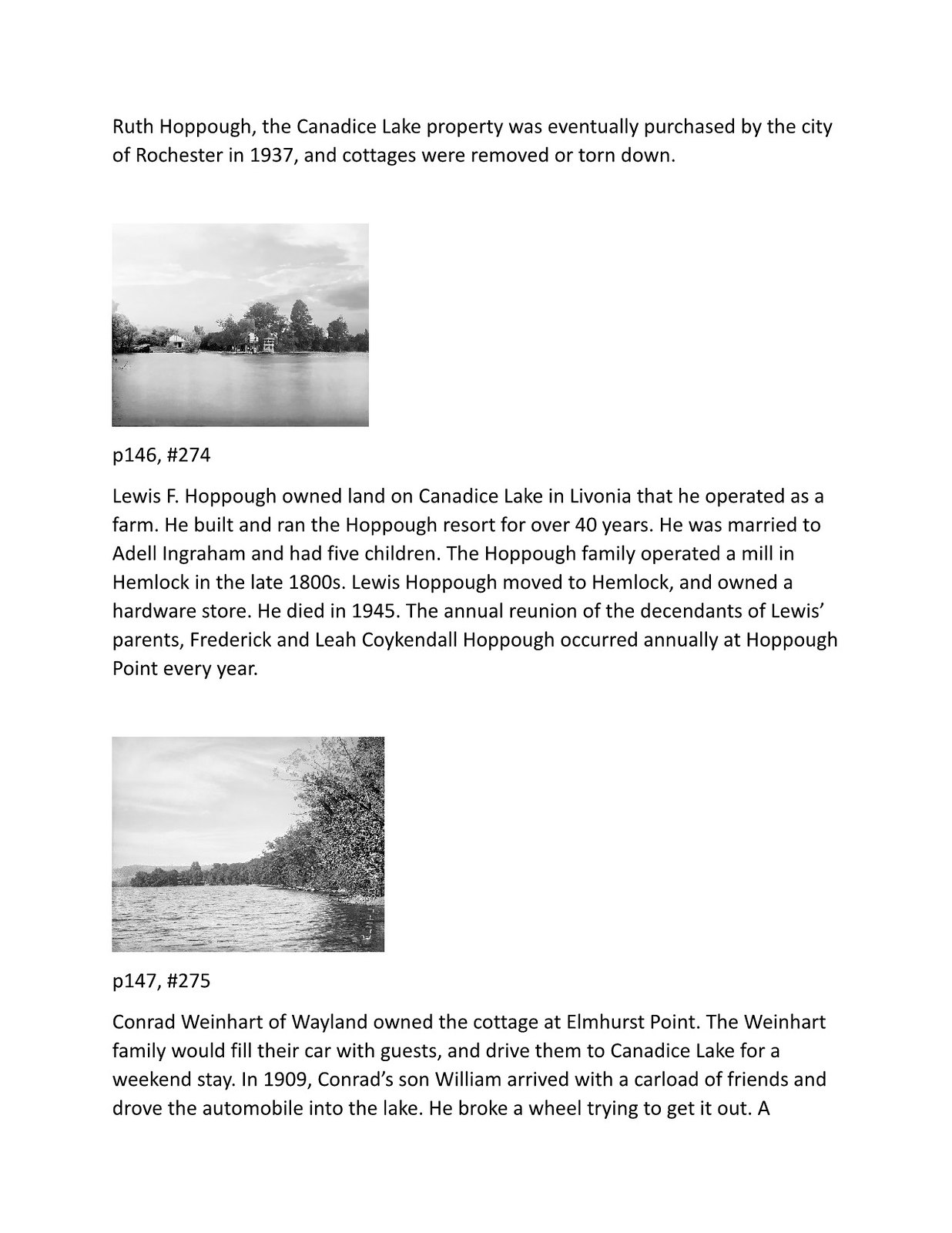The image appears to be an excerpt from an article, featuring two black-and-white photographs of Candence Lake. The upper photograph shows a view of the lake with cottages and trees lining the distant shoreline, accompanied by text reading, "Ruth Hoppo, the Candence Lake property was eventually purchased by the city of Rochester in 1937, and the cottages were removed or torn down." The caption also includes "P146, number 274," and describes how Louis F. Hoppo owned land on Candence Lake in Livonia, operated a farm, built, and ran the Hoppo Resort for over 40 years. He was married to Adele Ingraham and had five children. The Hoppo family operated a mill in Hemlock in the late 1800s, and Louis also owned a hardware store before his death in 1945. The annual reunion of the descendants of his parents, Frederick and Leah Kuykendall Hoppo, took place at Hoppo Point each year.

The lower photograph depicts another part of the lake with no visible properties, just trees, and shoreline. The accompanying text reads, "P147, number 275," and notes that Conrad Weinhart of Weyland owned the cottages at Elmhurst Point. The Weinhart family often drove guests to Candence Lake for weekend stays, and in 1909, Conrad's son William famously drove a car loaded with friends into the lake, breaking a wheel in the process. Additional text hints that more of the story continues on another page.